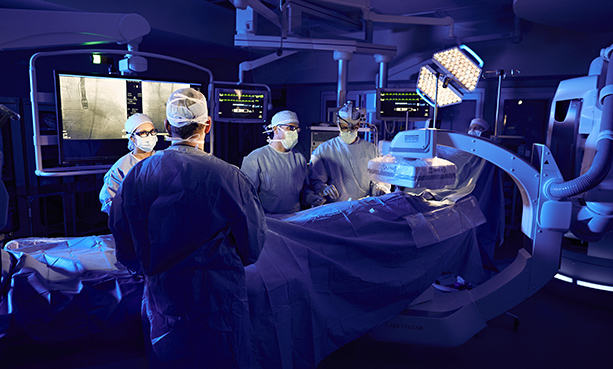In a dimly lit operating room, five medical professionals—four of whom are clustered around an operating table—are visible as they conduct what appears to be a surgical procedure. The patient, draped in a blue surgical sheet, is mostly obscured from view. The room is filled with an array of large medical equipment, including a ceiling-mounted light fixture and robotic devices. The doctors, nurses, and surgeons are all clad in protective gear: blue scrubs, face masks, surgical hats, and gloves. Various monitors in the background display vital signs in green text on black screens, with at least one screen likely showing a live feed of the procedure. The overall tone of the room is dominated by dark blues and violets, contributing to the focused and intense atmosphere of the surgical event.